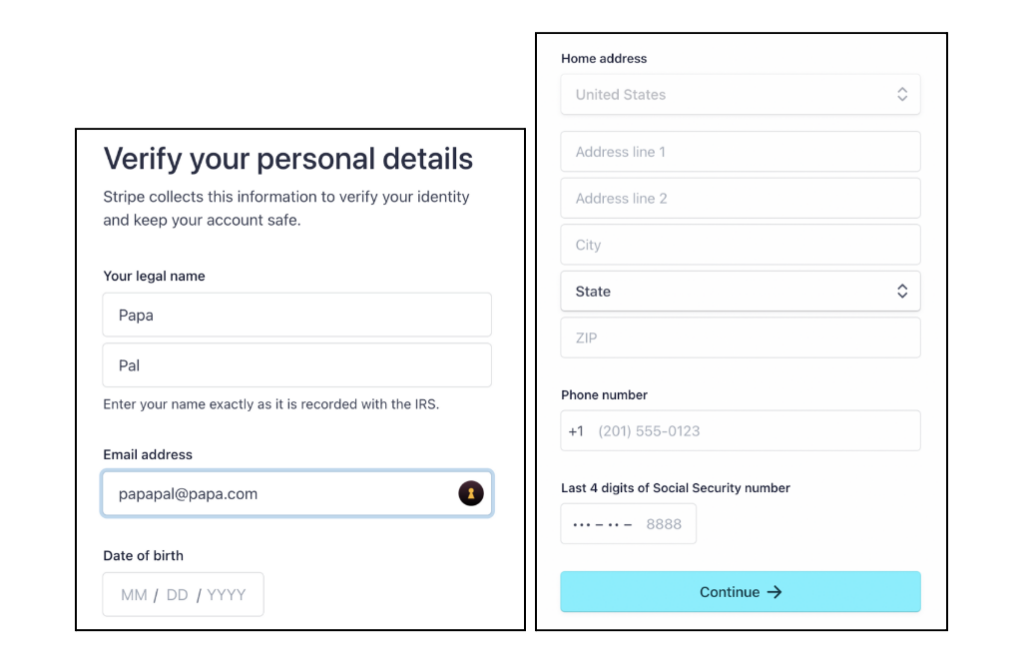The image consists of two side-by-side screenshots. The screenshot on the left is a square frame, while the one on the right is a rectangular frame. Both are distinct boxes containing form elements.

### Left Screenshot (Square Frame):
- **Title**: “Verify Your Personal Details”
- **Subtitle**: “Stripe collects this information to verify your identity and keep your account safe.”
- **Form Elements**:
  1. **Legal Name**: 
     - **Input Box**: “Papa”
     - **Subtext**: “pal”
     - **Instruction**: “Enter your name exactly as it is recorded with the IRS.”
  2. **Email Address**:
     - **Input Box**: “papapal@papa.com”
  3. **Date of Birth**:
     - **Input Box Placeholder**: “MM/DD/YYYY”

### Right Screenshot (Rectangular Frame):
- **Title**: “Home Address”
- **Form Elements**:
  1. **Country**:
     - **Input Box**: “United States”
  2. **Address Line 1**:
     - **Input Box**: [Blank]
  3. **Address Line 2**:
     - **Input Box**: [Blank]
  4. **City**:
     - **Input Box**: [Blank]
  5. **State**:
     - **Dropdown Menu**: [State Selection]
  6. **Zip Code**:
     - **Input Box**: [Blank]
  7. **Phone Number**: 
     - **Input Box Placeholder**: “Example: (123) 456-7890”
  8. **Last Four Digits of Social Security Number**:
     - **Input Box**: “88**” (Partial entry visible, cuts off)

At the bottom of the rectangular frame, there is a light blue bar stretching from left to right. On this bar, there is a darker blue button labeled “Continue” with an arrow pointing to the right.